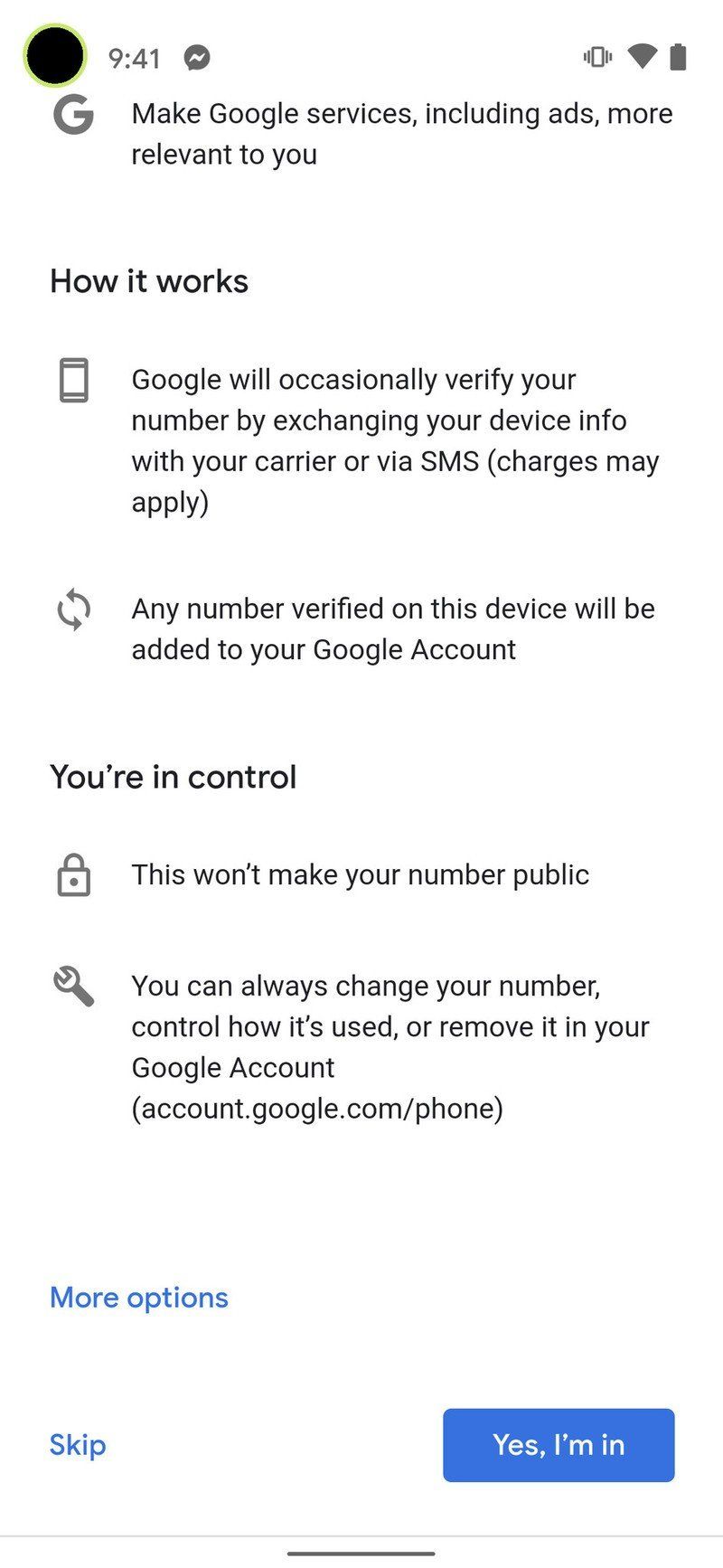The image is a screenshot of a Google service prompt aimed at making their services, including ads, more relevant by verifying the user's phone number. At the top left corner, the Google logo is prominently displayed, immediately above the main heading which states, "Make Google services, including ads, more relevant to you."

Below this heading, there are two main sections with corresponding headings and detailed explanations. The first section, titled "How it works," explains that Google will occasionally verify your phone number by exchanging device information with your carrier or via SMS, with a note that charges may apply. It also mentions that any number verified on the device will be added to your Google account. Accompanying this explanation are two icons: a phone icon next to the first point, and a circular arrow icon next to the second point.

The second section is titled "You’re in control." This section reassures users that verifying their number will not make it public. It emphasizes that users have control over their number, including the ability to change, control its usage, or remove it in their Google account settings.

At the bottom of the prompt, aligned horizontally, are two buttons: one labeled "Skip" and the other labeled "Yes, I’m in."

The overall layout is neatly organized, with each section clearly delineated by headings and supported by relevant icons for visual assistance.